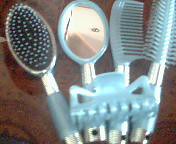This out-of-focus, low-resolution photograph showcases a set of hair grooming tools arranged on a patterned rug featuring shades of brown, tan, rust red, and orange. The image includes four main items, all matching in light blue and metallic silver, suggesting they are part of a cohesive set. From left to right, the items are as follows: a flat, round hairbrush with dark bristles tipped in white and a light blue grip on a metallic handle; a small oval hand mirror framed in light blue with a silver metallic handle; a blue comb with a silver handle; and another round hairbrush with blue bristles and a metallic handle. Additionally, a large light blue hair clip with interlocking teeth sits atop these tools, adding to the organized display.